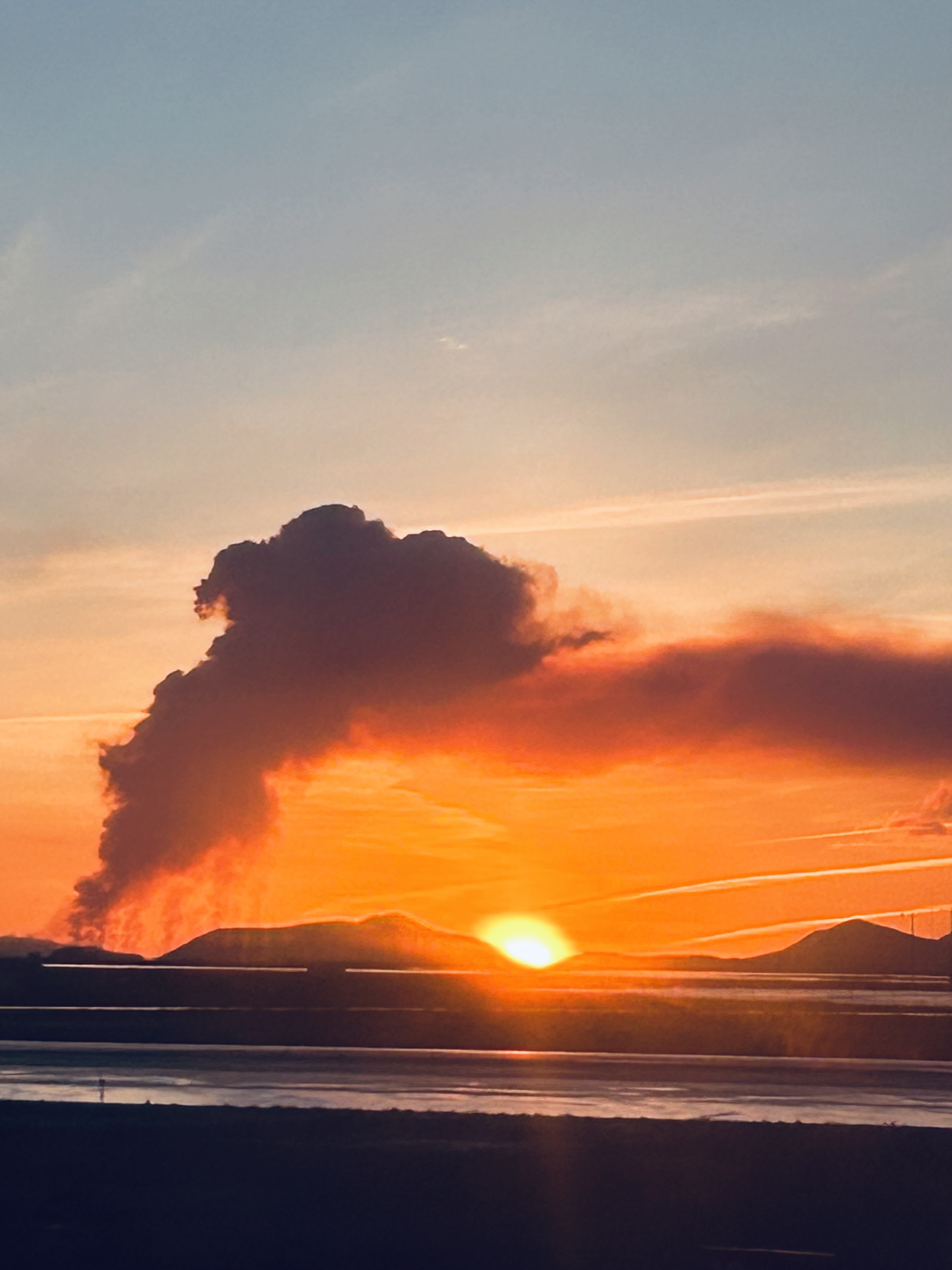In this stunning photograph of a sunset, the bright yellow sun is sinking into the horizon, illuminating the sky with a gradient of vibrant colors. At the top of the image, the sky transitions from a soft, pale blue to light orange near the horizon, with hues of dark orange and gray highlighting the dramatic scene. A dark gray, almost black, cloud hangs ominously overhead, and wisps of whitish-gray clouds scatter across the sky.

In the center of the frame, the setting sun is partially obscured by rolling hills or mountains, adding depth to the picturesque landscape. The lower portion of the image is notably darker, accentuating the striking contrast between the illuminated sky and the dim foreground. A line of dense black smoke, possibly from a fire or smokestack, rises from the lower left corner, intensifying as it ascends and adding a mysterious element to the scene.

In the foreground, a road with a guardrail can be seen, suggesting that the photograph was taken from a moving vehicle, which explains the motion blur at the bottom part of the image. The captivating composition captures the fleeting beauty of the sunset, blending natural serenity with an element of human activity.